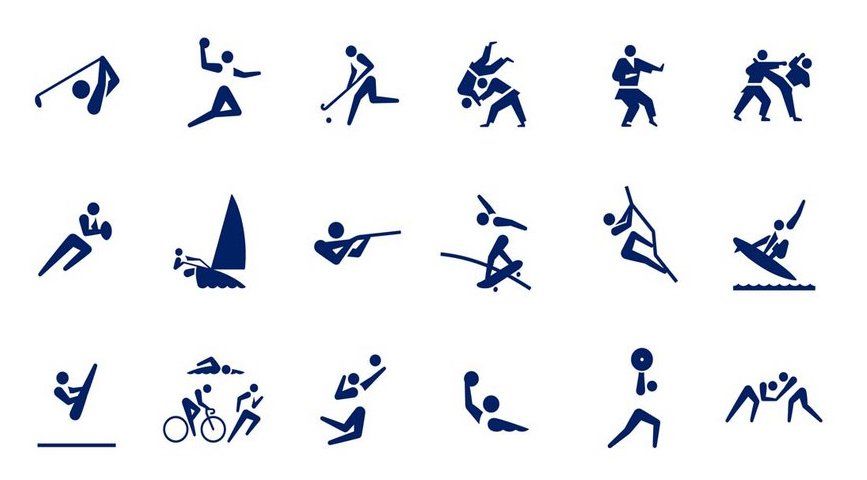The image features a collection of 18 blue, abstract stick figure icons, each representing a different sport. Arranged in a neat, evenly spaced 3x6 grid, these stylized illustrations depict various athletic activities. The first icon in the top left shows a golfer mid-swing, followed by a basketball player performing a dunk, and a field hockey player. Other sports include judo, with one figure flipping another, and a martial artist in a tai chi stance. Additional icons depict activities such as football, sailing, shooting, skateboarding, surfing, bike riding, running, volleyball, weightlifting, and wrestling. The icons are simply outlined and placed one next to another without borders, all set against a white background, suggesting a possible theme of Olympic events.